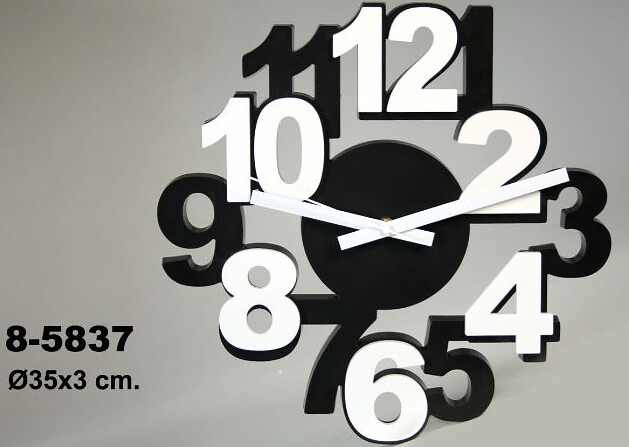The image is wider than it is tall and features a modernistic clock positioned on the right-hand side. The clock's numbers are artistically floating, with the numerals 12, 2, 4, 6, 8, and 10 prominently displayed in white against a black backdrop, while the numbers 1, 3, 5, 7, 9, and 11 appear in black and are subtly positioned behind the white numbers. At the center of the clock, the minute and hour hands are represented as sleek white rectangles that contrast sharply against a black circle, which seems to be placed in the middle of the white and black layers of the numbers 12, 2, 4, 6, 8, and 10. On the lower left-hand side of the image, there are black numerals inscribed as "8-5837," along with a null sign, and dimensions noted as "35x3 centimeters." The overall background of the image is a gradient of gray and white, adding depth and a minimalist touch.